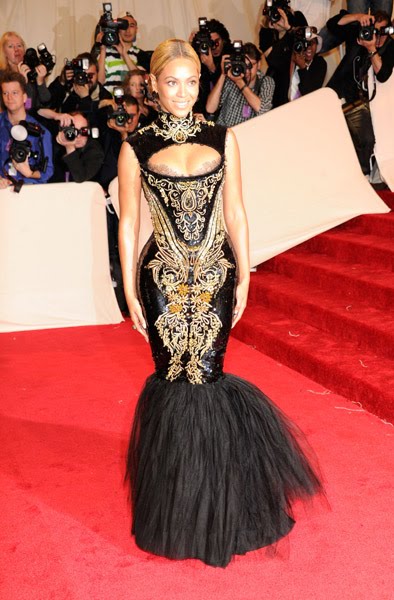In this vibrant outdoor scene, Beyoncé is captured on a red carpet at a glamorous event, possibly a premiere or gala. She stuns in an elegant black and gold sleeveless gown, featuring intricate gold floral trims along the torso and neck. The dress has a distinctive circular cutout at the bosom, and cascades into a fluffy, tutu-like, ruffled section from the knees down, extending past her feet. Beyoncé's golden hair is tied back, highlighting her radiant smile as she poses for the cameras with one arm relaxed by her side. Behind her, a backdrop of a white barrier separates her from a throng of paparazzi armed with cameras and camcorders, eager to capture her every move. Adjacent to her, a striking red staircase complements the red carpet, completing the regal atmosphere of the scene.